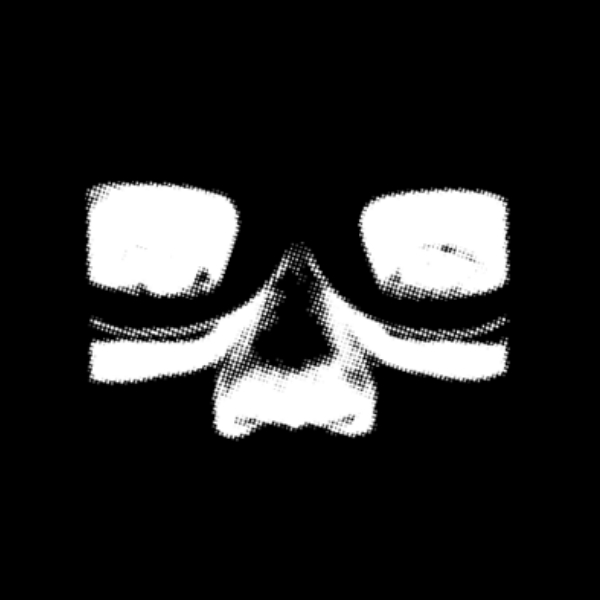This black and white graphic image, featuring a pixelated effect formed by small black dots, presents a close-up of a person's face. The composition is from a perspective slightly below the subject, looking up at their face. Prominently depicted are the black glasses with indistinguishable white spaces inside, resembling the effect of sunglasses or an x-ray with a rectangular-like shape. The image faintly outlines the eyes and detailed shading of the nose, with black shading tapering to gray near the nostrils and along the sides of the nose. Only the section from above the eyes to just below the nose is visible, with the rest of the face obscured by darkness, giving it an impression of a partial portrait. The face appears to have a full nose, potentially indicating it might be an x-ray image of someone who could have had a broken nose, adding to the abstract yet detailed nature of this black and white artwork. The background is meticulously squared off with black, emphasizing the defined space around the face, further enhancing the mysterious and intricate effect of the image.